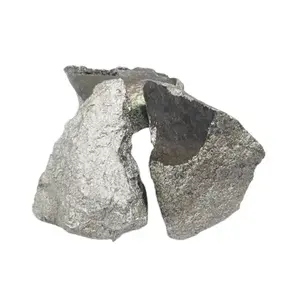The image features two prominent stones against a plain white background. The stone on the right is a combination of two shades of grey: a lighter, metallic-looking grey at the bottom and a darker, flat grey forming a V shape at the top. The stone has irregular, uneven edges and divots at its base. On the left, the stone is lighter, with a silvery grey base transitioning into a darker grey towards the top, which appears to connect seamlessly with the stone on the right, separated by a narrow gap resembling the opening of a large keyhole. A third, triangular-shaped stone resides in the background, characterized by its darker, shaggier appearance. The foreground stones, when viewed together, have been likened to the shape of a lung, with the top portions appearing smooth while the bottom parts show rough, bumpy textures.